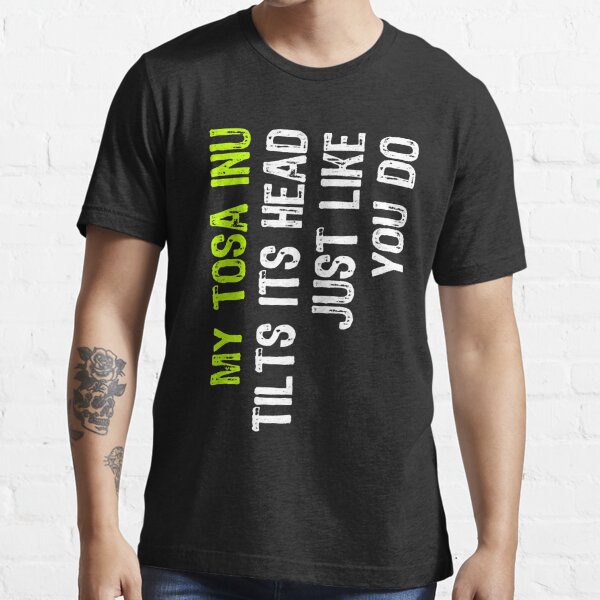The photograph depicts a Caucasian individual from the neck to the waistband, standing against a bright, almost washed-out white brick wall. The person is wearing a gray, short-sleeved, round-necked t-shirt with distinctive writing printed sideways from the bottom to the top on the left side. The bold green text reads: "My Tosa Inu," followed by smaller white text stating, "tilts its head just like you do." The individual’s right arm features a tattoo of a skull with a flower emerging from it, along with two other tattoos partially visible and wrapping around the back of the arm. The person is also dressed in blue jeans, with their arms resting down at their sides.